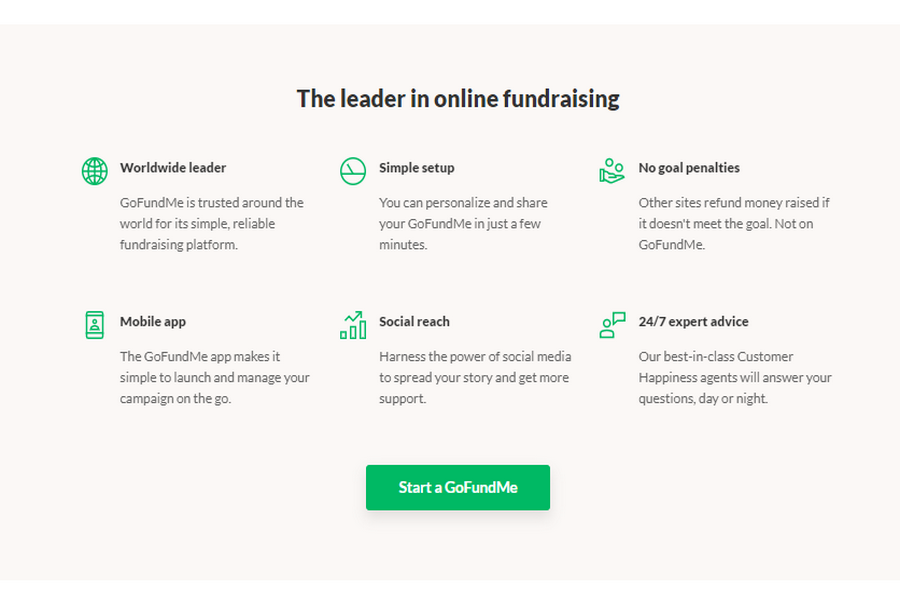**Caption:**

The image highlights GoFundMe as "The Leader in Online Fundraising" in bold, black text at the top. It showcases six key features organized in a grid with three rows and two columns against a light gray background.

- **Top Left: Worldwide Leader**
  - *Description:* GoFundMe is trusted around the world for its simple, reliable fundraising platform.

- **Top Right: Mobile App**
  - *Description:* The GoFundMe app makes it simple to launch and manage your campaign on the go.

- **Middle Left: Simple Setup**
  - *Description:* You can personalize and share your GoFundMe in just a few minutes.

- **Middle Right: Social Reach**
  - *Description:* Harness the power of social media to spread your story and gain more support.

- **Bottom Left: No Goal Penalties**
  - *Description:* Other sites refund money raised if it doesn't meet the goal, but not with GoFundMe.

- **Bottom Right: 24/7 Expert Advice**
  - *Description:* Our best-in-class customer happiness agents are available to answer your questions day or night.

At the bottom, a green rectangle with white text invites users to "Start a GoFundMe."